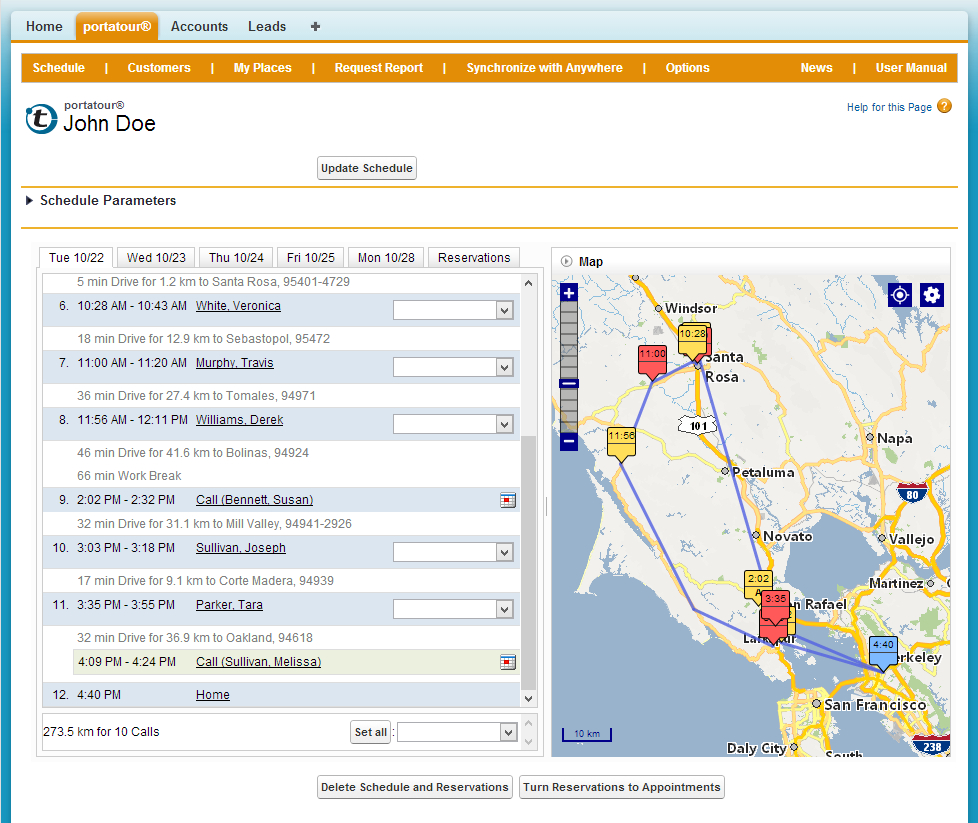**Detailed Descriptive Caption:**

The image features a user interface with a structured layout. At the top-left corner, several tabs are displayed, including "Home," "Portal Tower," "Account," and "Lit." The "Portal Tower" tab is highlighted in orange, while the others are written in black. Below this top section, there's a secondary menu with tabs labeled "Schedule," "Customer," "My Places," "Request," "Reports," "Synchronize with Anywhere," "Options," "News," and "User Manual." These tabs are written in white against an orange background.

On the left side, beneath the secondary menu, the user's profile area is displayed, showing "Portal Tower" and the user name "John Doe," accompanied by a blue circle icon with the letter "T" inside. In the center of the interface, a prominent button labeled "Update Schedule" is visible.

To the left of the button, a section titled "Schedule Parameters" lists various schedule entries organized by date. The dates include "Tuesday 10, 2022," "Wednesday 10," "Thursday 10," "Friday 10," and "Monday 10, 28." Below these dates, reservations are listed starting from number 6 at 10:28 AM to 10:43 AM, marked as "white, Veronica." The sequence continues with numbers 7 through 12. At the bottom of this section, it states "273.5km for 10 calls," indicating the total distance covered for 10 scheduled calls. There are empty drop-down menus next to each entry, suggesting additional customizable options.

On the right side of the image, a detailed map is displayed. The map features blue areas representing water, yellow and orange lines indicating roads and main roads. Additionally, there are blue icons at the top right of the map for "Current Location" and "Settings."

At the bottom of the image, two grey and black buttons are present, labeled "Delete Scheduled Reservation" and "Send Reservation to Appointments." These options allow further interaction with the scheduling interface.